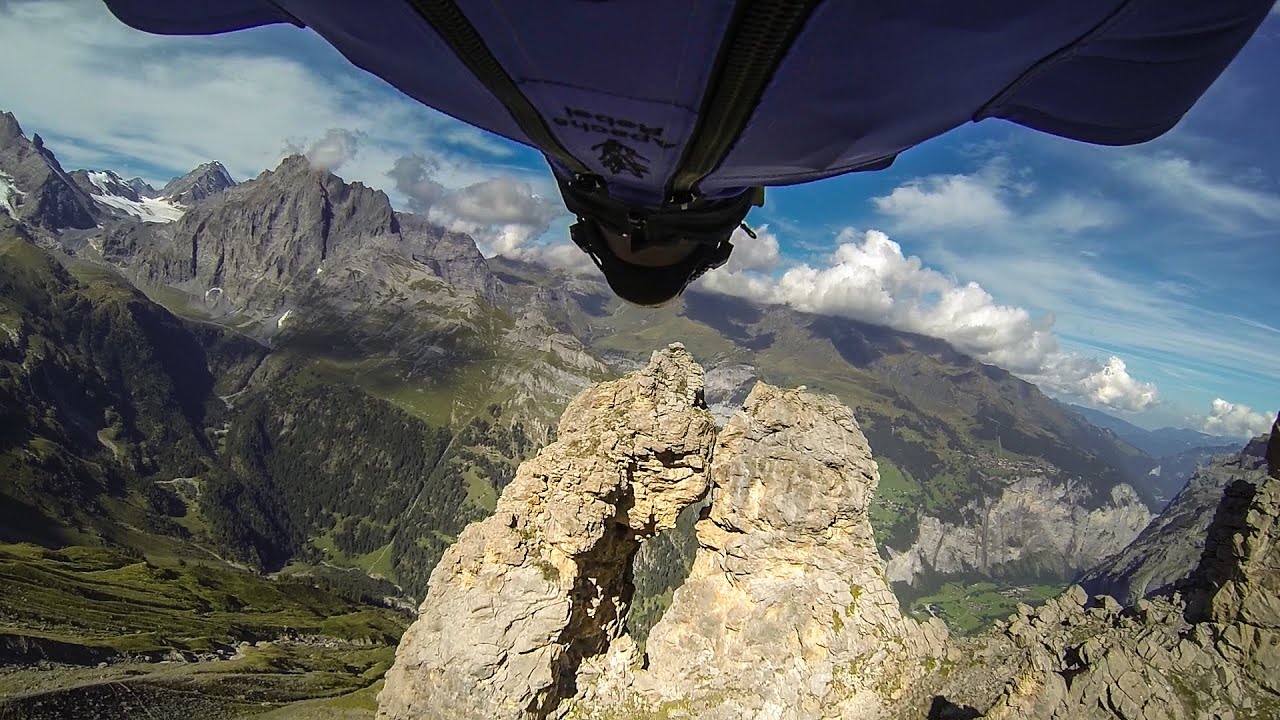This detailed aerial photograph captures a breathtaking mountainous landscape. The image appears to be taken from a camera mounted on the body of a person wearing a distinct outfit. At the top of the image, a person in a blue vest with black lettering and gold zippers is partially visible, including the bottom of their chin, suggesting that they are wearing a helmet and the camera is on their body. The foreground showcases a prominent yellowish rock structure while the background features a vibrant green valley filled with vegetation. To the left, the rugged mountains are coated with trees at lower elevations and some snow at higher peaks. Above, the sky is beautifully blue, scattered with white clouds, creating a picturesque and ethereal view. The overall scene exemplifies the convergence of rugged natural beauty and human exploration.